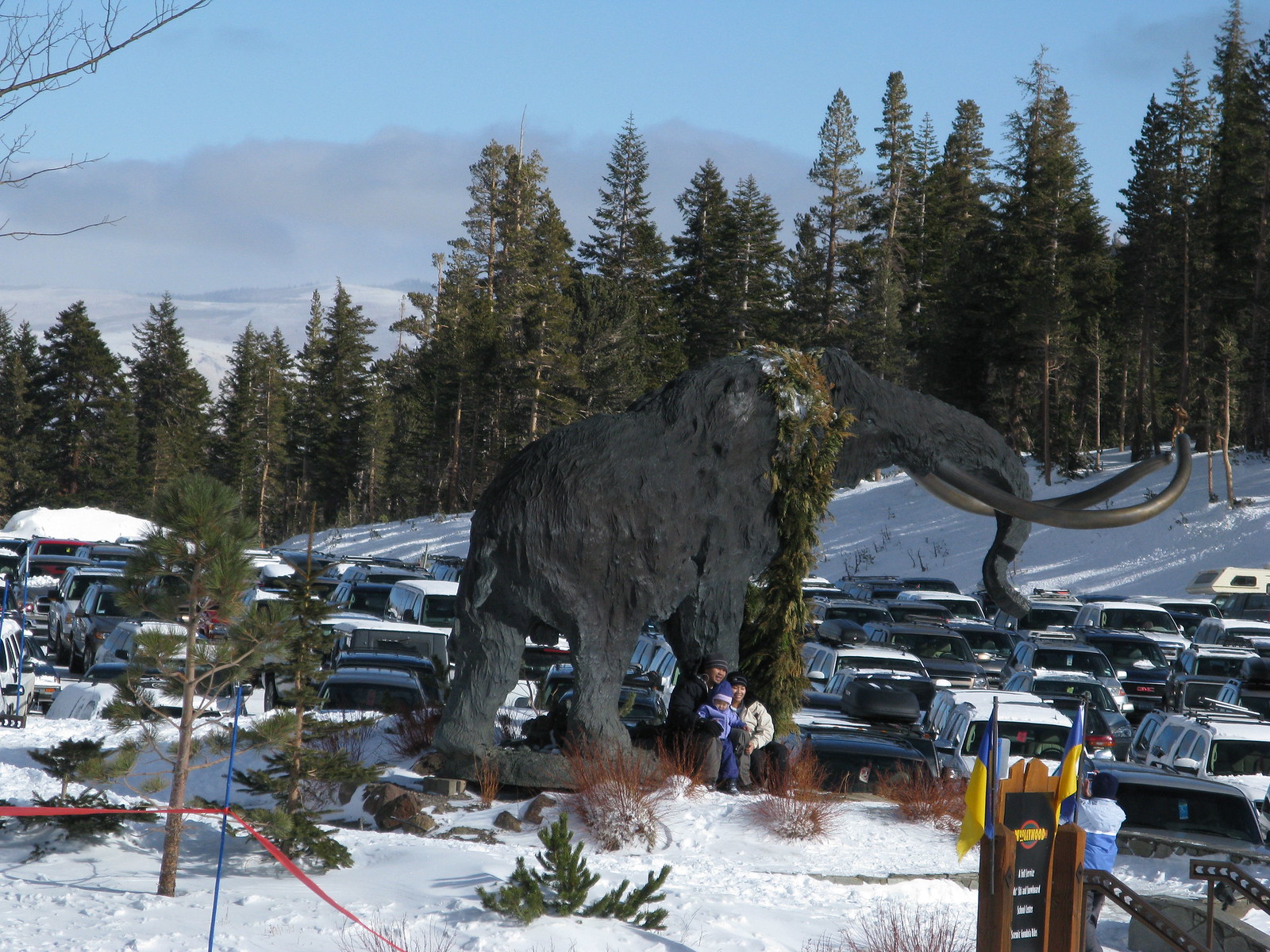The image captures a snowy scene featuring a large gray statue of a woolly mammoth prominently placed in a bustling, snow-covered area, possibly a popular camping or skiing destination. The mammoth is adorned with green vines draped over its head and is facing right. In front of the statue, three Asian individuals—a man, a woman, and a baby—are posing for a photograph taken by another person standing in the bottom right corner. Surrounding this scene is a large parking lot filled with cars blanketed in snow. The backdrop includes a snowy hill rising to the right, covered with dense, dark green pine trees that stretch across the image. Beyond the trees, mountains and clouds are visible under a light blue sky, adding to the picturesque winter landscape.